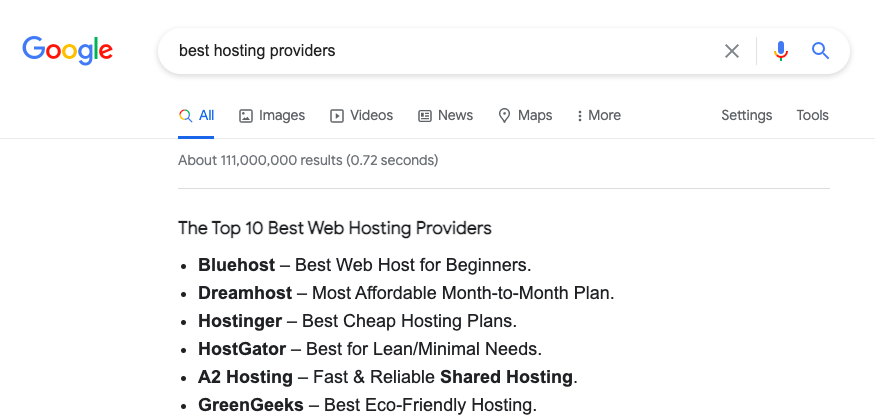The image depicts a Google search results page. At the top left, the Google logo is prominently displayed. To its right is a search bar, flanked by two icons on the far right side, with a gray 'X' mark within the text field. The text within the search bar reads: "Best Hosting Providers". Just below, there is a horizontal navigation menu with multiple categories; the "All" category, situated at the far left, is highlighted in blue text and underlined, indicating it is the selected filter. Further down, the page reveals that there are approximately 111,000,000 results generated in less than 0.75 seconds. The search results showcase a list of top web hosting providers, with their names in bold. The listings include:
- **Top 10 Best Web Hosting Providers**
- **Bluehost** - Best Web Host for Beginners
- **DreamHost** - Most Affordable Month-to-Month Plans
- **Hostinger** - Best Cheap Hosting Plans
- **HostGator** - Best for Lean, Minimal Needs
- **A2 Hosting** - Fast and Reliable Shared Hosting
- **GreenGeeks** - Best Eco-Friendly Hosting